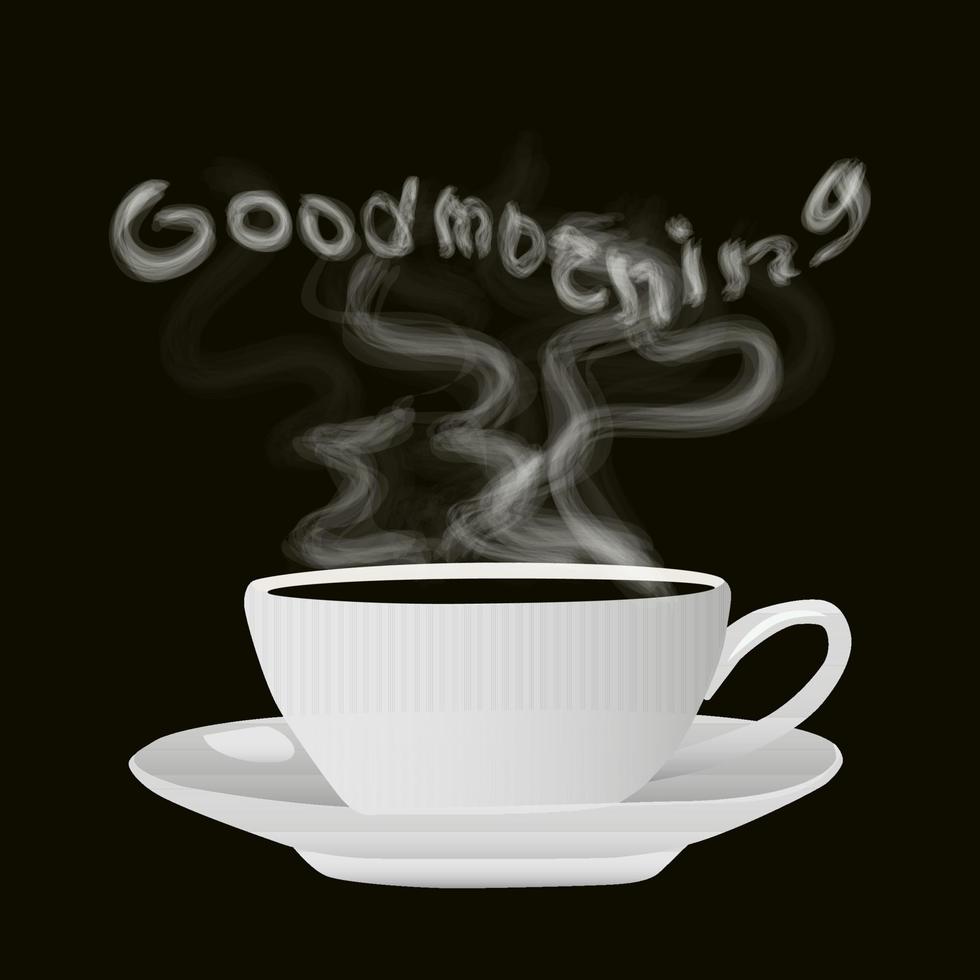The image is a highly detailed, computer-generated artistic rendering of a white coffee mug with a matching white saucer, set against a completely black background. The mug, which has a shallow design with simple reflections on its handle and the saucer's edge, contains a dark liquid. Halfway up the mug, there's a pattern of vertical lines. From the hot coffee rises white steam that swirls upward, shaping the light gray-white words "Good Morning" in a rough, slightly see-through font. The glossy surface of both the mug and the saucer adds to the polished, realistic yet somewhat cartoonish aesthetic of the image.